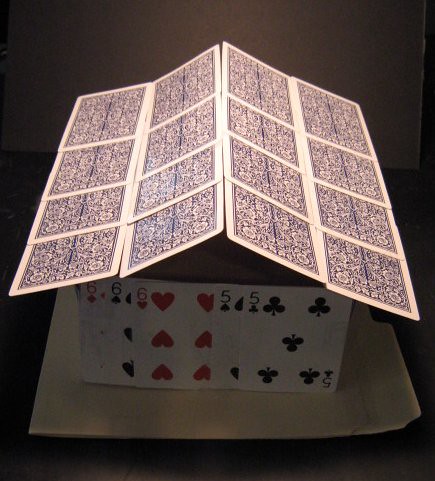In this meticulously constructed image, a literal "house of cards" is featured, built atop a dark brown, possibly black, wooden tabletop. Dominating the lower section of the scene is a manila file holder, its beige hue muted by shadows cast across it. Rising from the tabletop, playing cards are arranged to form the walls and roof of the card house. The roof is composed of four slanted playing cards, each bordered in white and adorned with a blue mosaic design akin to traditional Bicycle playing cards.

The front wall of the card house is artfully arranged with several specific cards: a six of diamonds, six of clubs, six of hearts, and a five of clubs paired with a five of spades. These cards stand upright, meticulously balanced to support the structure. Above them, an intentional triangular gap creates an airy void at the roofline. The background of the scene is a solid gray wall, contrasting subtly with the dark tabletop and the brighter elements of the card house. The lighting in the image is focused primarily on the roof, lending a dynamic shadow play that enhances the three-dimensional illusion of this fragile yet compelling construction.